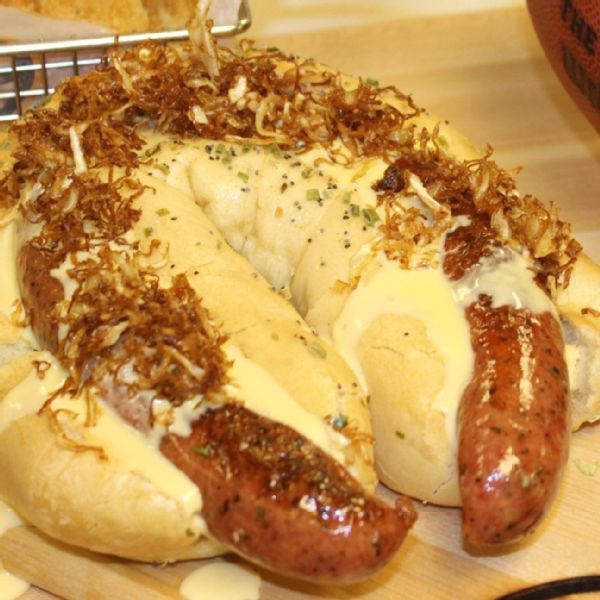The image showcases a thick, seasoned kielbasa baked into a horseshoe-shaped, cheesy bread. The golden-brown kielbasa prominently emerges from the bottom of the loaf, while white cheese oozes around the baked sausage. Encircling the kielbasa, thin onion strips follow the same horseshoe pattern, adding texture and flavor. In the background, a silver barred dish is partially visible, covered by the substantial bread loaf. The entire composition rests on a rustic wooden table, contributing to the homey ambiance of the scene.